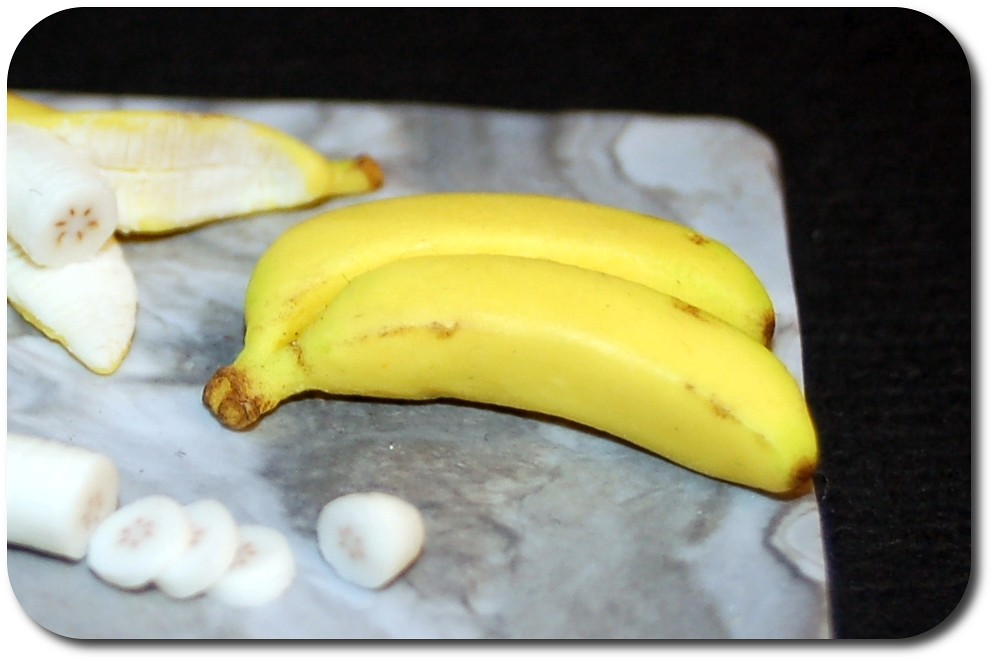A vibrant photograph captures three bananas in perfect clarity. Two whole, yellow bananas are joined at the stem, showcasing their unblemished skins. In the background, another banana—peeled to reveal its creamy white flesh—rests nearby. This banana has been partially sliced, with neatly cut, round pieces prominently displayed in the foreground. All of this is set against a richly textured marble or granite surface, speckled with shades of brown, gray, and white. The entire scene is framed within a larger, darker background, emphasizing the illuminated countertop and its contents, while obscuring any surrounding details. The bananas are pristine, with minimal bruising, emphasizing their freshness.